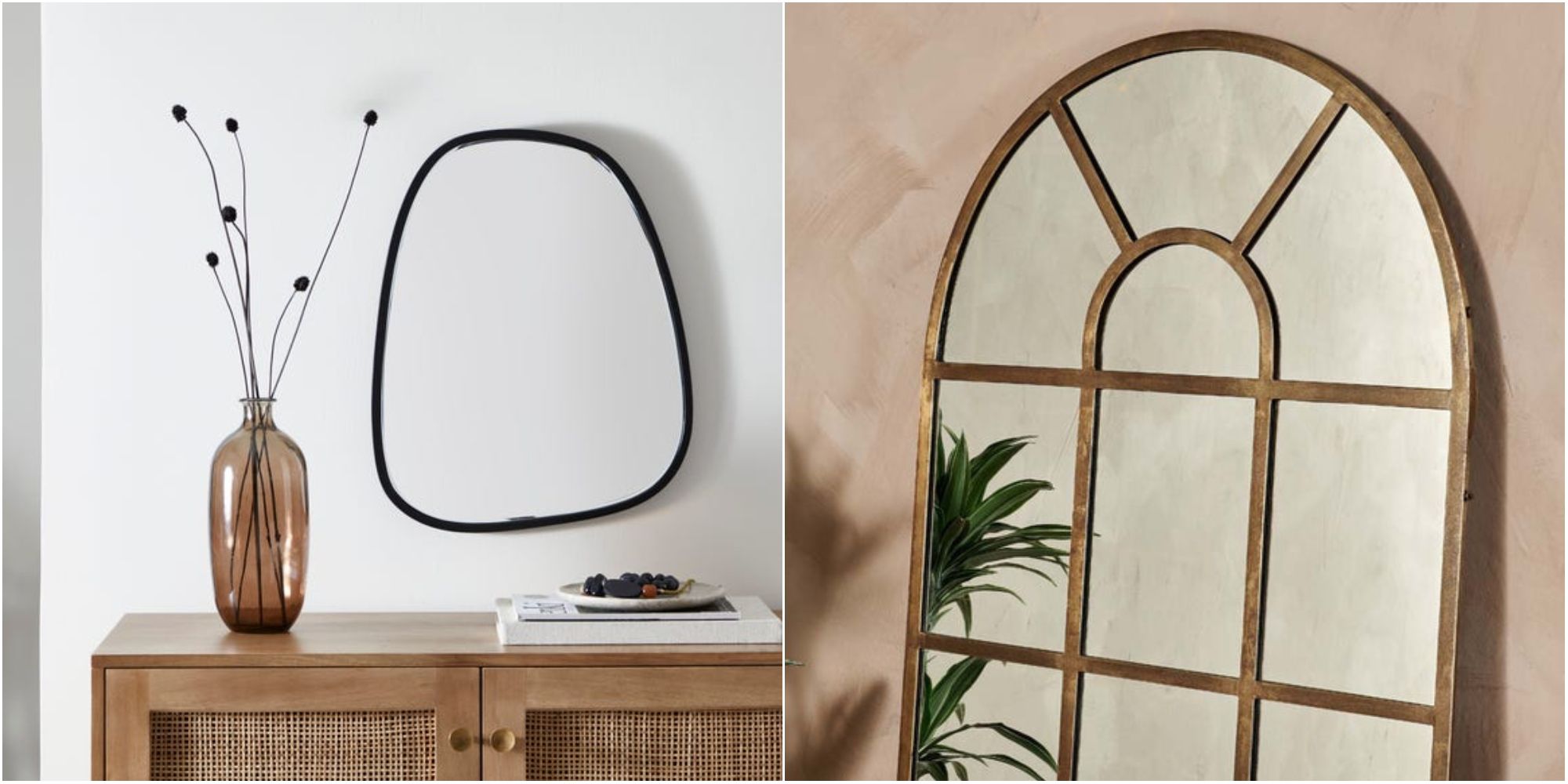The image set consists of two side-by-side photographs likely sourced from a catalog, possibly for home furnishings. The left image features a white-walled room with a short, light-wood console adorned with two large doors that have woven fronts. Atop this console stands an amber-colored, oval-shaped vase about a foot tall, containing six long, black stems that end in small balls. Adjacent to the vase is an oval-ish, irregularly shaped mirror hanging on the wall. The console also holds a pair of books with a plate of berries resting on top. In the second, close-up photograph, a large, arch-shaped mirror with an ornate brass frame stands against a peach-beige wall, displaying visible paint strokes. The frame is detailed with various gold lines forming a geometric pattern, giving the impression of multiple mirrors. The reflection in the mirror includes the image of a potted houseplant, adding a touch of greenery to the scene.